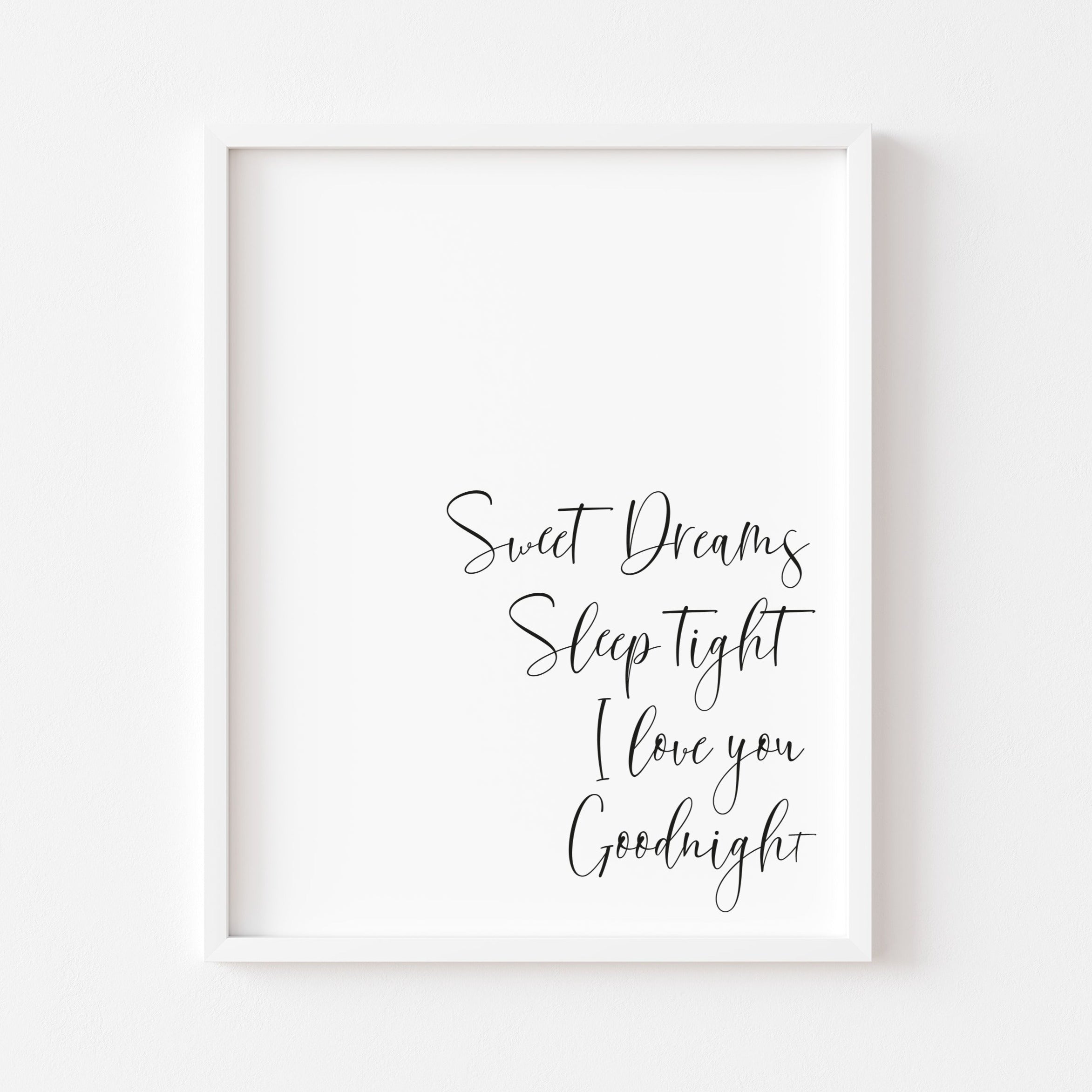The image predominantly features white hues, creating a clean and minimalist aesthetic. At the center of this bright white photograph or realistic AI rendering, there is a white frame or potential shadow box hanging on a white wall. This frame casts subtle shadows both on its interior and exterior, suggesting a soft light source originating from the top left. Inside the frame, on a stark white canvas, resides a four-line text in a loose, handwritten script—a blend of cursive and print—located in the bottom right quadrant. The text reads: "Sweet dreams, sleep tight, I love you, good night," with specific capitalization on "Sweet," "Dreams," "Sleep," "Tight," "I," "Love," and "Good." Around 70% of the image is negative space, emphasizing the simplicity and elegance of the handwritten message. The overall design resembles decor items commonly found in retail stores like Target, suitable for a living room or a bedroom.